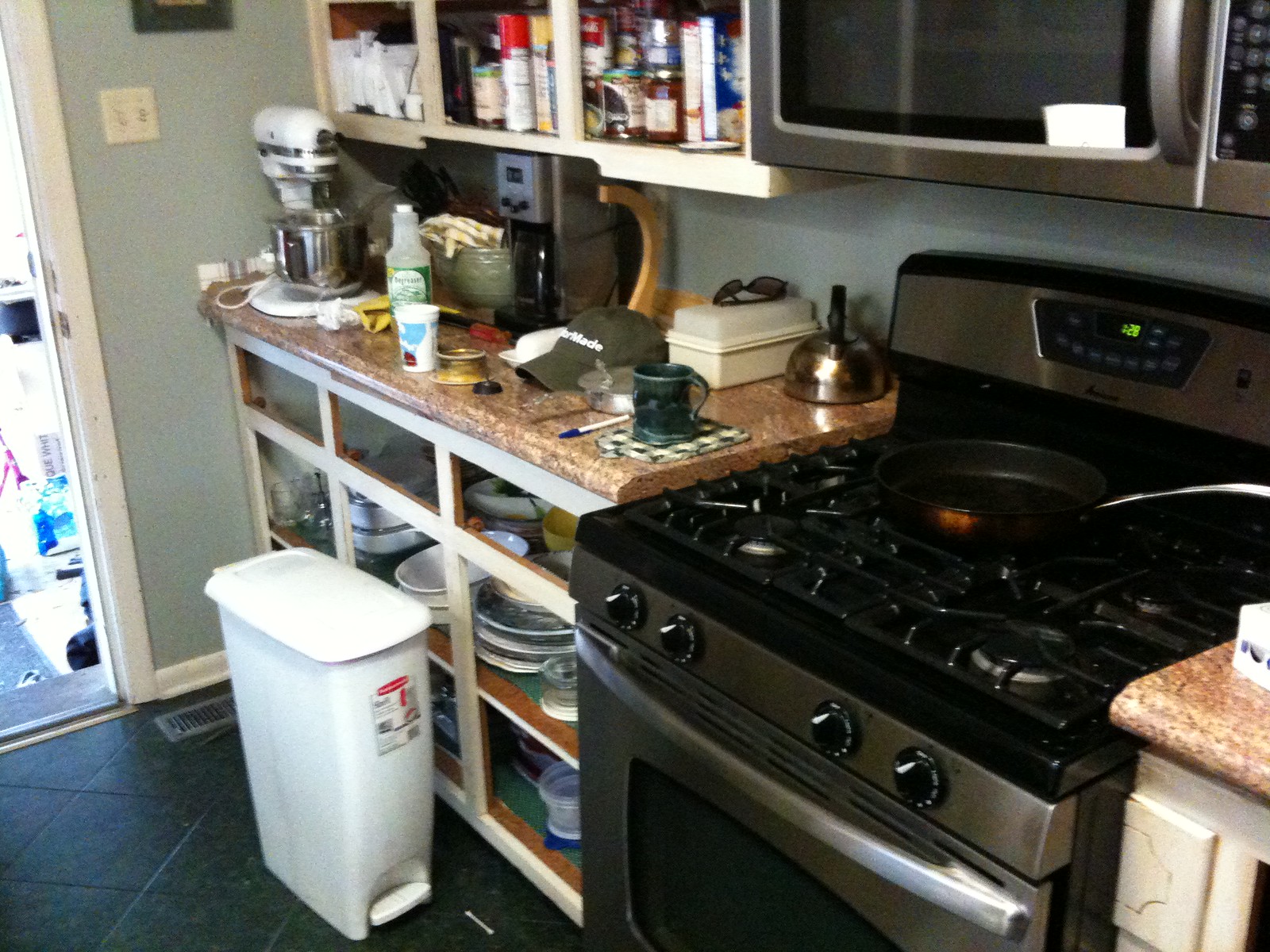The photograph captures a section of a modern EV kitchen. Central to the image is a black and gray stove, prominently featuring a pan in the middle of the stovetop. Above the stove, a coordinated gray and black microwave is mounted, seamlessly blending with the kitchen's sleek design. Flanking the stove on either side is a counter topped with luxurious brown and tan marble. The counter, however, is missing drawers, making the plates and cups stored inside visible. An assortment of items is scattered on the countertop: a green mug resting on a coaster, a pen with a blue cap, and a white container topped with a pair of black sunglasses. Adjacent to the counter is a white trash can, discreetly positioned at the edge of the scene.